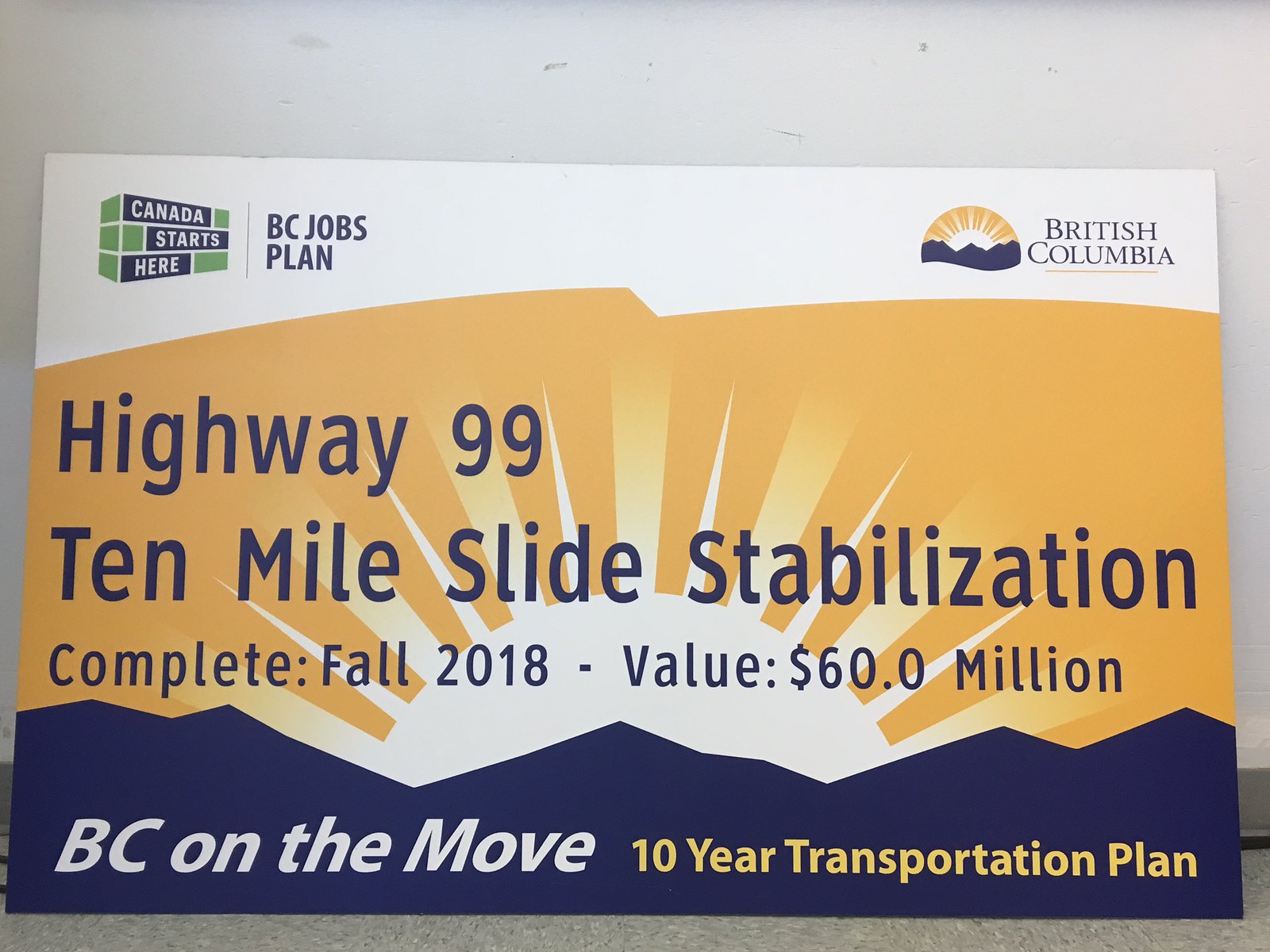The image features an informational sign set against an off-white or light beige background. Central to the image is a card-like sign positioned directly in the middle. The sign prominently displays multiple elements: 

- In the top left corner, there is a blue logo with the text "Canada Starts Here" followed by "BC Jobs Plan" in smaller white letters.
- In the top right corner, a logo for British Columbia is present, accompanied by the text "British Columbia."
- Below this, against a beige background with blue lettering, it reads "Highway 99, 10 Mile Slide Stabilization."
- Further down, the text states "Complete: Fall 2018," and "Value: $60,000,000."
- Towards the bottom, set against a blue drawn mountain range, it reads "BC On The Move" in white lettering, followed by "10 Year Transportation Plan" in yellow.

The color scheme incorporates gray, white, dark blue, green, yellow, orange, and purple, emphasizing the informational and formal nature of the sign as part of a program or transportation plan announcement. The overall style of the sign is corporate and informational, likely related to a government transportation project.